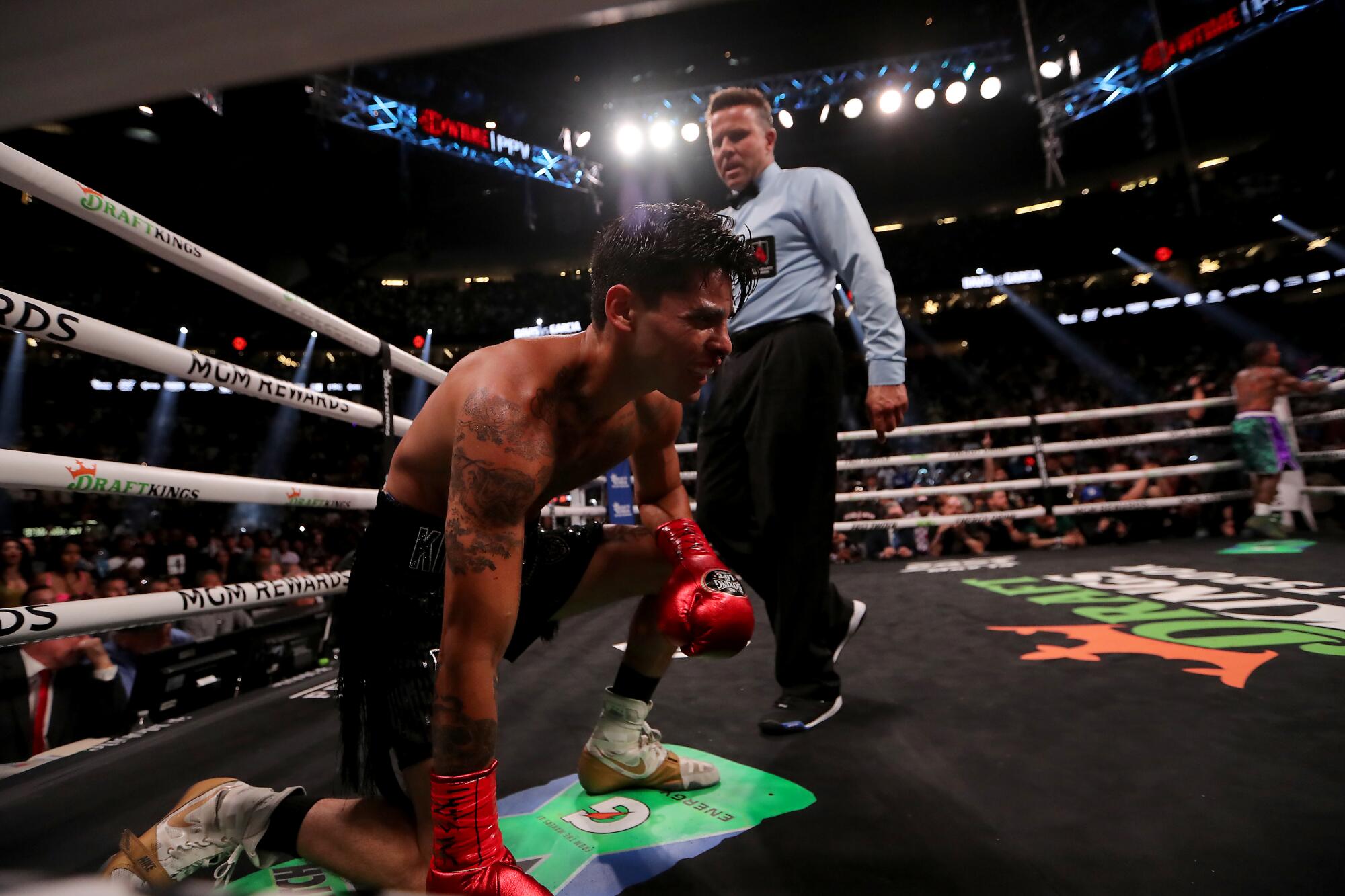The photograph captures an intense moment inside a well-lit, crowded arena. At the center-left of the image, a shirtless, tattooed boxer with curly black hair and likely of Hispanic descent is kneeling on one knee, appearing hurt. He wears red boxing gloves, black shorts, and white Nike high-top sneakers. His left arm rests on his other knee, and he is positioned on a black canvas adorned with Gatorade logos and a DraftKings symbol. To his right stands a referee in dark pants, a long-sleeve blue shirt, and a black bow tie, attentively watching the downed fighter. In the background, the other boxer, wearing greenish-blue shorts, is seen in his corner. The boxing ring is surrounded by white ropes displaying "MGM Rewards" and "DraftKings" logos, with a cheering crowd and dazzling lights completing the backdrop.